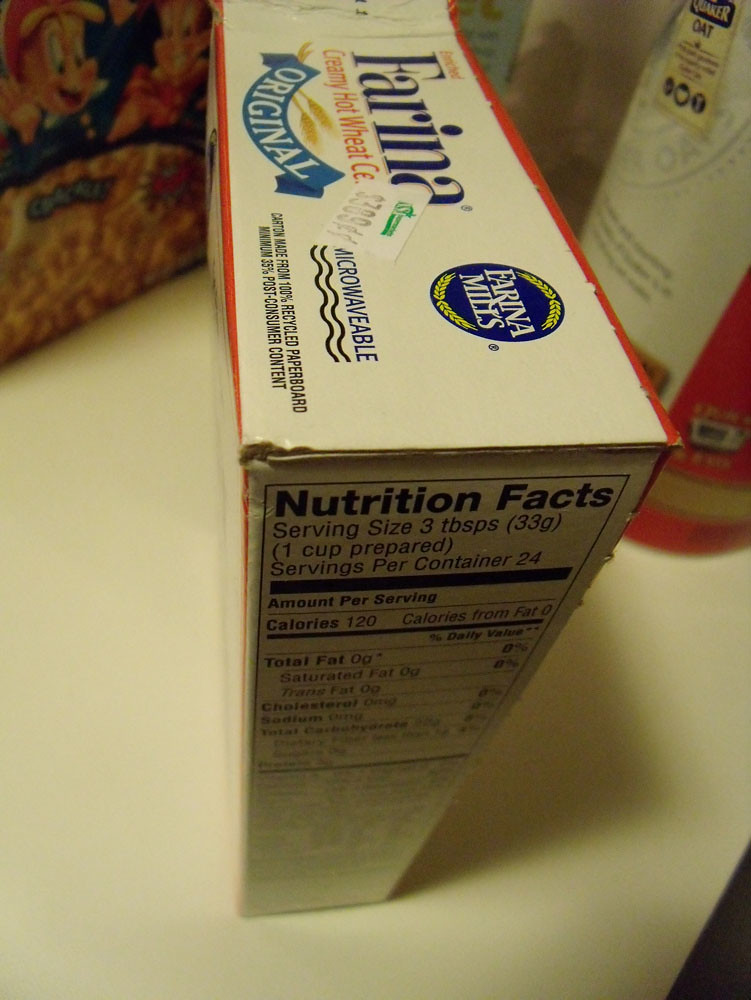The photograph displays a contemporary still-life of groceries, prominently featuring a tall, rectangular cardboard box in the foreground. The box is labeled "Farina Original Creamy Hot Wheat Cereal" by Farina Mills, with both the top and the nutrition facts side of the box clearly visible. A price tag can also be spotted on the box. Emerging from behind the Farina box is a partial view of a round, red-and-white container, though the rest of it is obscured and its contents remain unidentified. To the left, there is a box of macaroni and cheese, identifiable by a cartoon fish illustration, suggesting it is a kid-friendly product. All three items are displayed on a clean, white countertop.